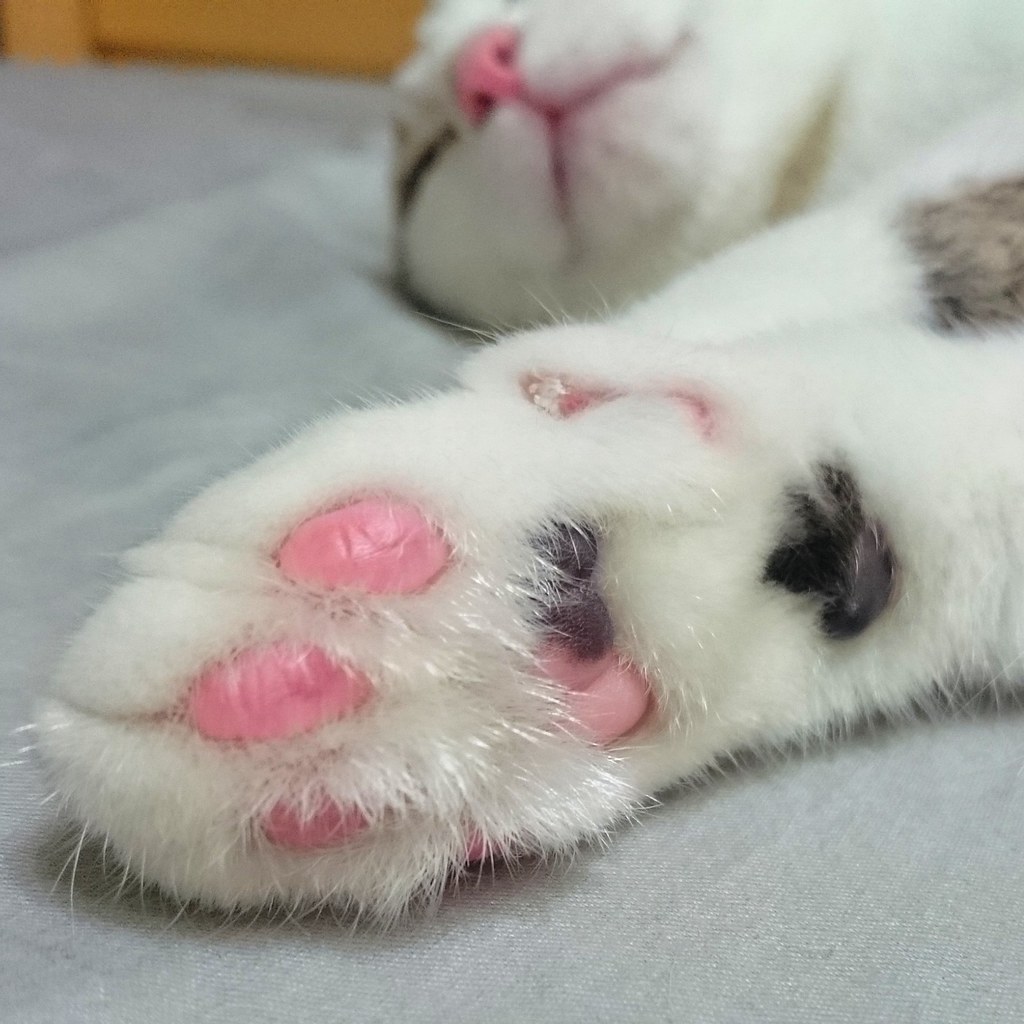This image captures a detailed close-up of a sleeping cat's paw and its head, which is slightly blurred in the background. The cat is lying on its right side on a silvery-gray fabric. Its white paw, which stretches from the right to the left side of the frame, has pink toe pads and a base pad that is half pink and half black. The short-haired fur on the paw is predominantly white, with a patch of light brown tabby fur and a bit of black visible near the tips. The cat's face, featuring a bright pink nose, and a triangular pink outline around the mouth, is partially visible. The eyes are closed, showing black slits, and the fur on its face, chin, and chest is white. The overall composition highlights the soft textures and contrasting colors of the cat's features against the gray background.